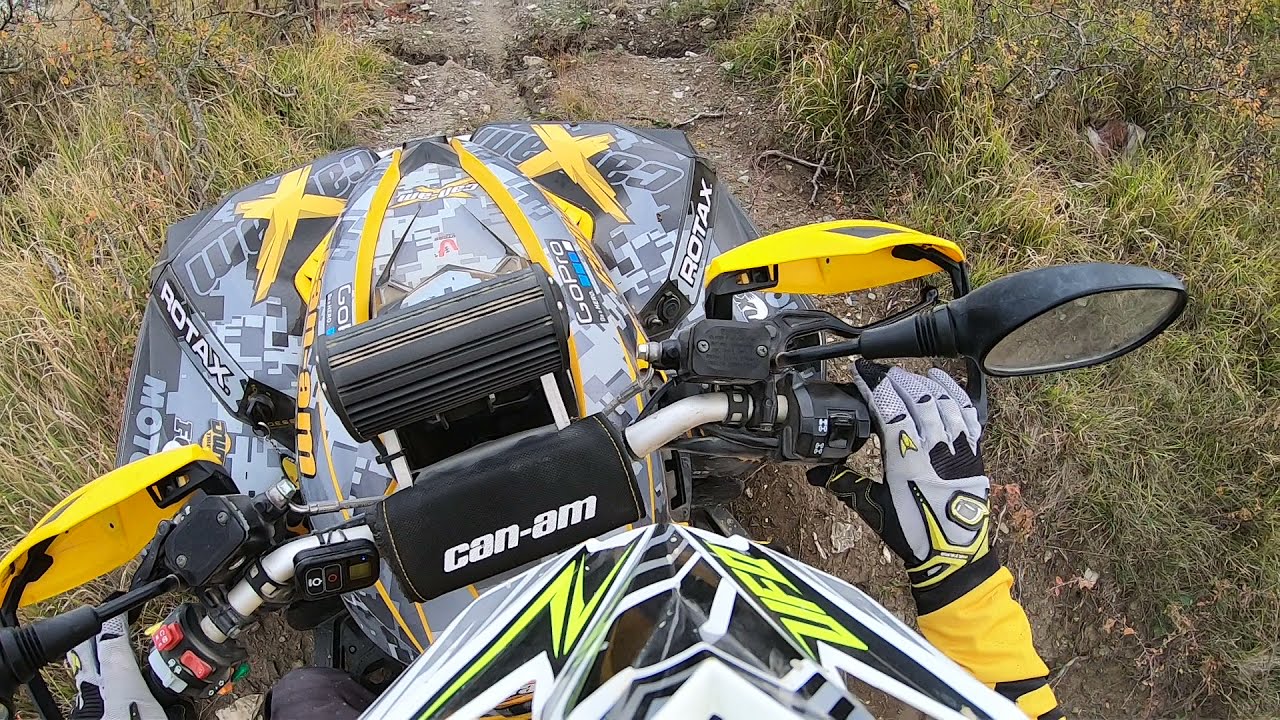This detailed caption integrates information from each of the voices to provide a comprehensive description of the image:

The image, captured from a GoPro camera mounted on top of a rider's helmet, shows the view from the perspective of someone riding an all-terrain vehicle (ATV). The ATV is predominantly colored in white, black, gray, and yellow, featuring a distinctive glitchy pattern with yellow accents. The person operating the ATV is dressed in a motocross outfit consisting of gloves and a yellow long-sleeve riding suit, matching the color scheme of the vehicle. The helmet, visible at the bottom of the image, is white, black, and yellow.

The handlebars of the ATV include shield protectors in yellow and a pad in the middle that reads "CAN-AM," confirming the vehicle's brand. The handlebars are black and gray, and there's a side-view mirror indicating additional detail. The terrain below consists of a dirt path flanked by grass and rocky patches, with green and brown colors prevalent in the background. There's also a small GoPro symbol visible on the right side of the ATV, reaffirming the perspective of the photo. This vibrant scene paints a lively picture of off-road adventure on a well-equipped four-wheeler.